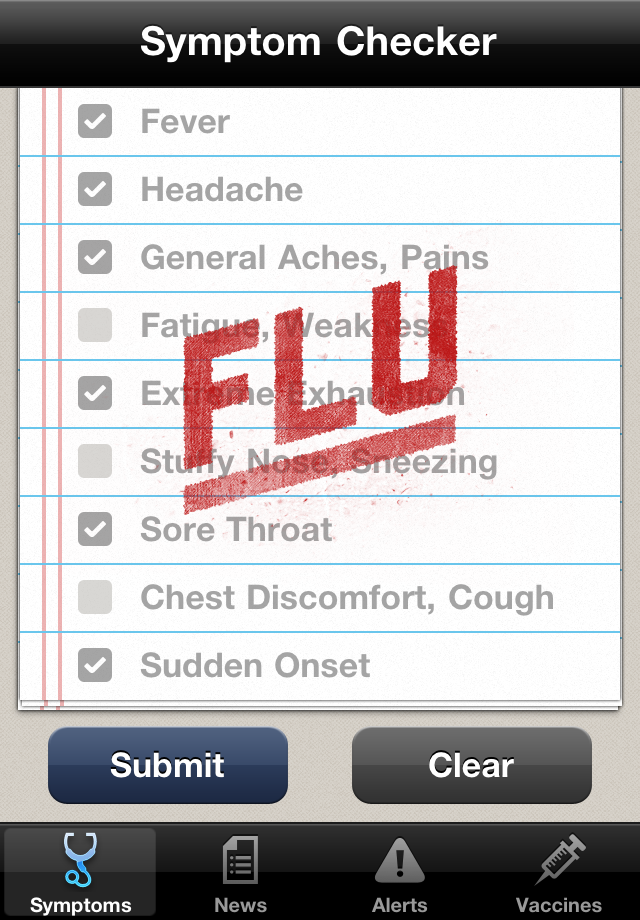This image appears to be a screenshot from a digital symptom checker app, possibly on a cell phone or tablet, designed for diagnosing the flu. At the top, there is a thick black header with "Symptom Checker" written in white text featuring a capital 'S' and 'C'. Below this, the main section resembles a digital lined notebook page, complete with blue horizontal lines and two thin red vertical lines on the left margin.

In the main body, a checklist of flu symptoms is displayed, including: Fever, Headache, General Aches and Pains, Fatigue and Weakness, Extreme Exhaustion, Stuffy Nose, Sneezing, Sore Throat, Chest Discomfort, Cough, and Sudden Onset. The symptoms that are checked off include Fever, Headache, General Aches and Pains, Extreme Exhaustion, Sore Throat, and Sudden Onset. Each symptom is listed in gray text with a corresponding checkbox to the left, which turns white when checked.

Centrally, the word "FLU" is prominently stamped in large red, uppercase letters at a diagonal angle, underlined for emphasis. This red label partially covers some of the symptoms: the 'F' intersects with "Fatigue," "Extreme," and "Stuffy," while the 'U' overlays the end of "Pains" and extends into "Weakness" and "Exhaustion."

Below the list, there are two buttons: a blue "Submit" button on the left and a gray "Clear" button on the right, both with white text. At the bottom of the screen, a black navigation bar features four icons: a highlighted blue stethoscope labeled "Symptoms," an icon of a newspaper labeled "News," a caution triangle with an exclamation point labeled "Alerts," and a syringe symbol labeled "Vaccines."